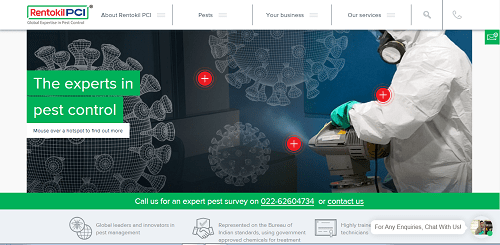This is a detailed caption for an image of a screenshot taken from a website:

"The screenshot displays a webpage from the brand Rentokyo PCI, prominently featuring several options at the top of the page, including 'About Rentokyo PCI.' The second option is unreadable, but additional options visible are 'Your Business,' 'Chat Services,' a 'Search' button, and a 'Call' button. Centrally located on the page is a photograph of an individual clad in an exterminator's outfit, showcasing their professional appearance. To the left of the image, a bold headline states, 'The Experts in Pest Control.' Beneath this headline, contact information is provided: 'Call us for an expert pest survey on 022 6260 4734 or contact us.' Although there are additional words at the bottom of the screenshot, they are too small to discern. The entire image maintains a rectangular shape, with no further distinct elements noted."